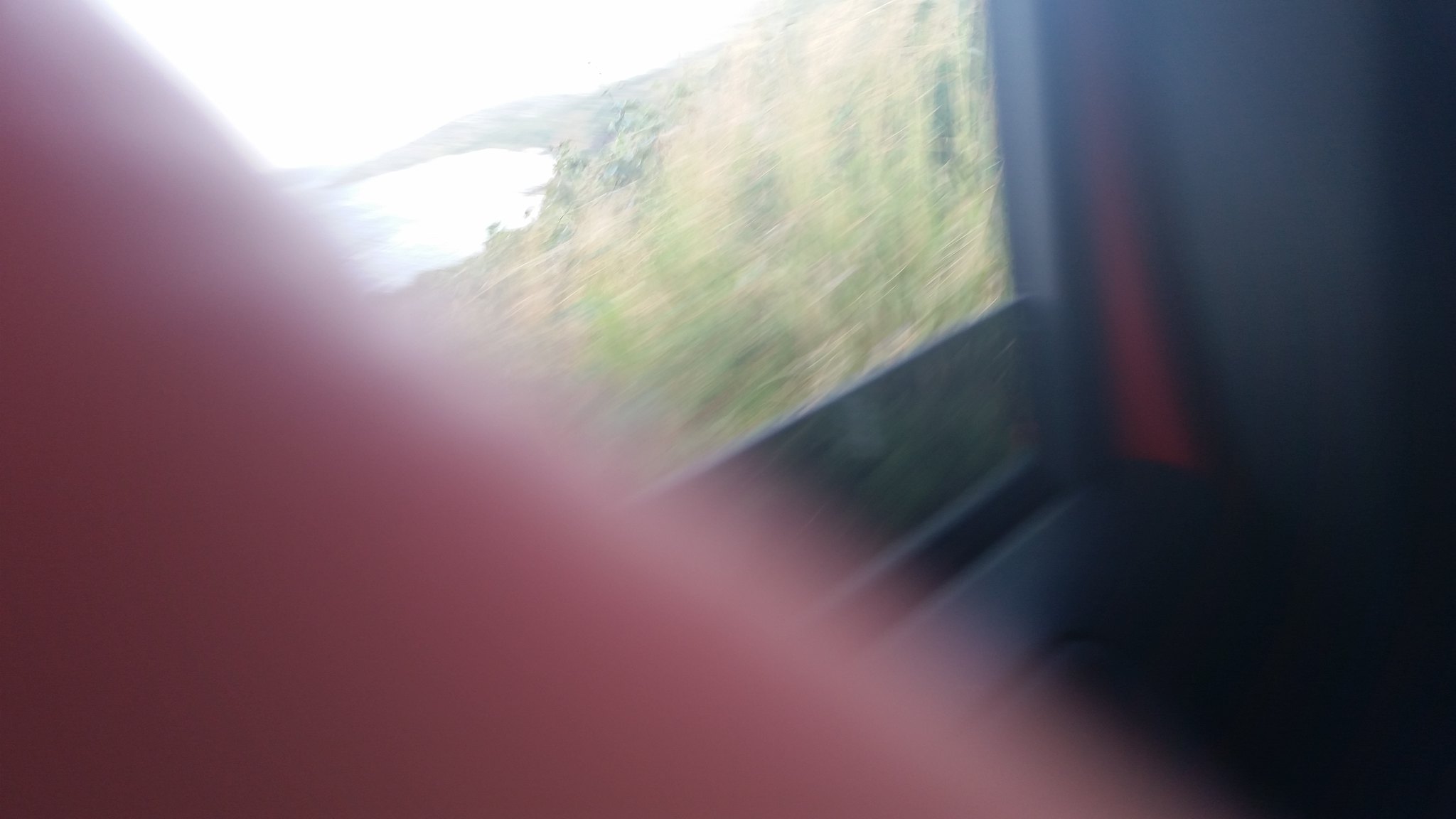This photograph, taken from inside a room looking out through a window, features a blurred overall image with the prominent interruption of a Caucasian finger crossing diagonally from the upper left corner to the bottom center of the horizontal frame. The window, framed in white, reveals an exterior view abundant with lush greenery and what appears to be a large, expansive lake under a white sky. Inside the room, the visible interior includes an ambiguous object placed in the corner to the right of the window. This object, mostly dark in color, extends downward towards the floor and is equipped with a brown handle. The combination of external and internal elements creates a layered composition, though the image's clarity is compromised by the prominent blur and finger obstruction.